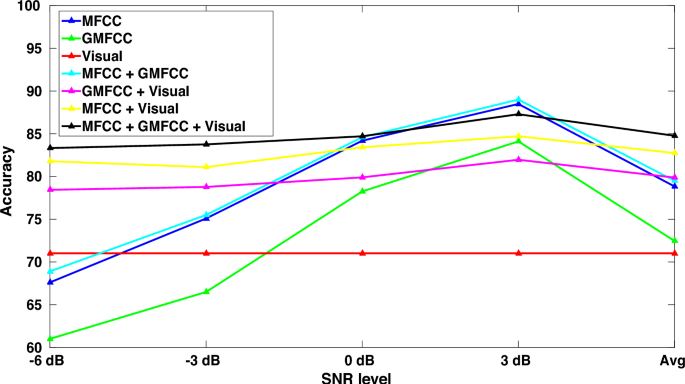This is a color image of a line graph, which is enclosed in a gray rectangular border. The vertical axis on the left side is labeled "Accuracy" with black text, and it ranges from 60 at the bottom to 100 at the top. At the top of the graph, there is a guiding header also in black text.

In the upper left-hand corner, there is a legend within a smaller gray box. The legend uses black text to indicate different line colors representing "MFCC" and "GMFCC," though their meanings are not specified. The graph features several colored lines representing data trends, some of which exhibit both upward and downward movements.

A red line prominently stands out, marking the accuracy level at approximately 72. The horizontal axis at the bottom of the graph is labeled "SNR Level" and is centered. The SNR (Signal-to-Noise Ratio) levels range from -6 dB, 0, to 3 dB. On the right side of the graph, there is an additional label that reads "ABG" or "Average," providing a summary metric for comparison.